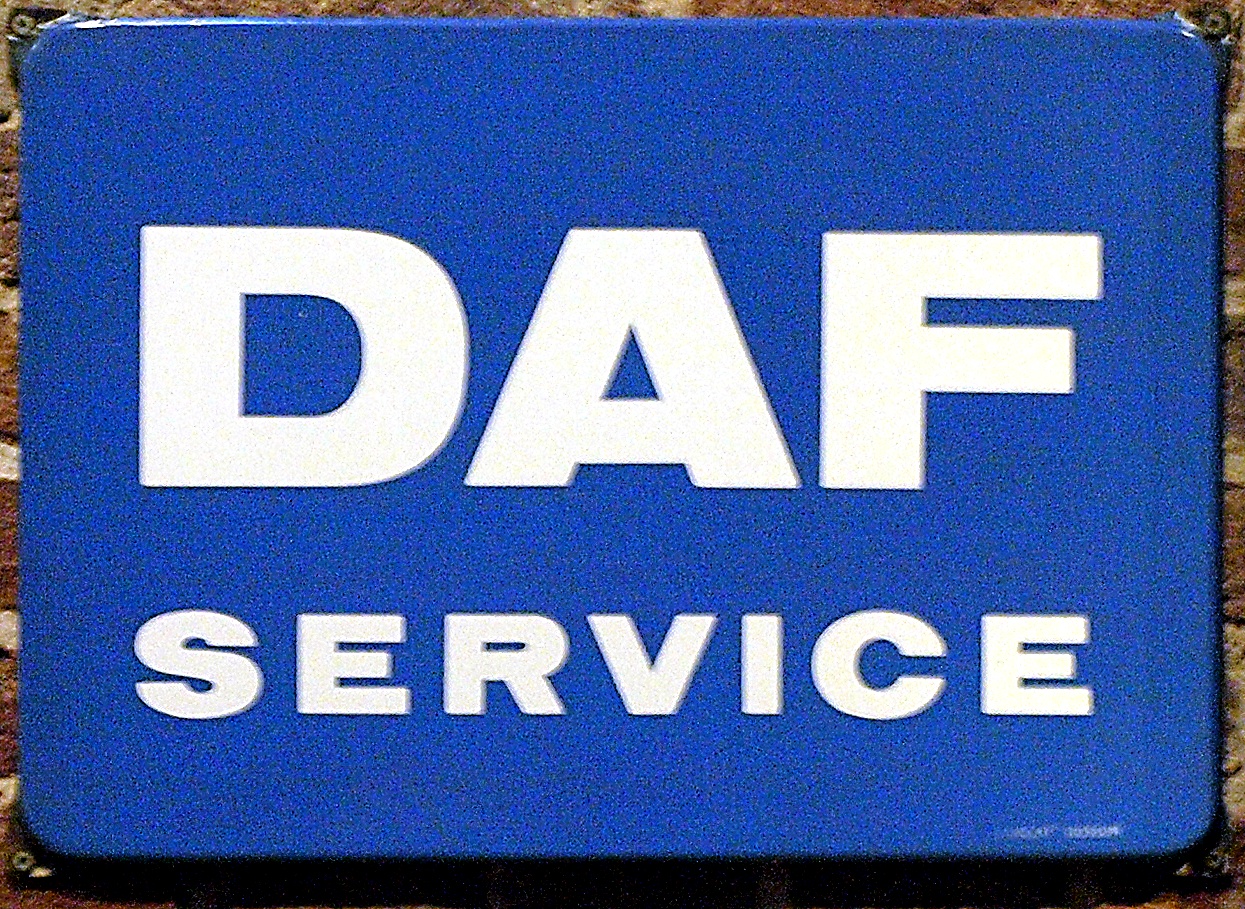In this image, there is a rectangular sign with rounded edges affixed to what appears to be a brick wall, although only a narrow, slightly visible border of red brick is seen due to the graininess of the photo. The sign is secured at each corner with screws, indicating its permanence. The body of the sign features a bright blue background heavily speckled with darker, black grainy spots due to the image quality. Centered on the blue background, white lettering stands prominent and clear despite the graininess. The text "D-A-F" is displayed across the top in large, bold, evenly spaced letters. Below, in slightly smaller, yet equally striking letters, the word "SERVICE" is spelled out, aligning perfectly beneath the top text, maintaining the same meticulous spacing. Despite the grainy quality of the picture, the essential details and the message of the sign are conveyed effectively.